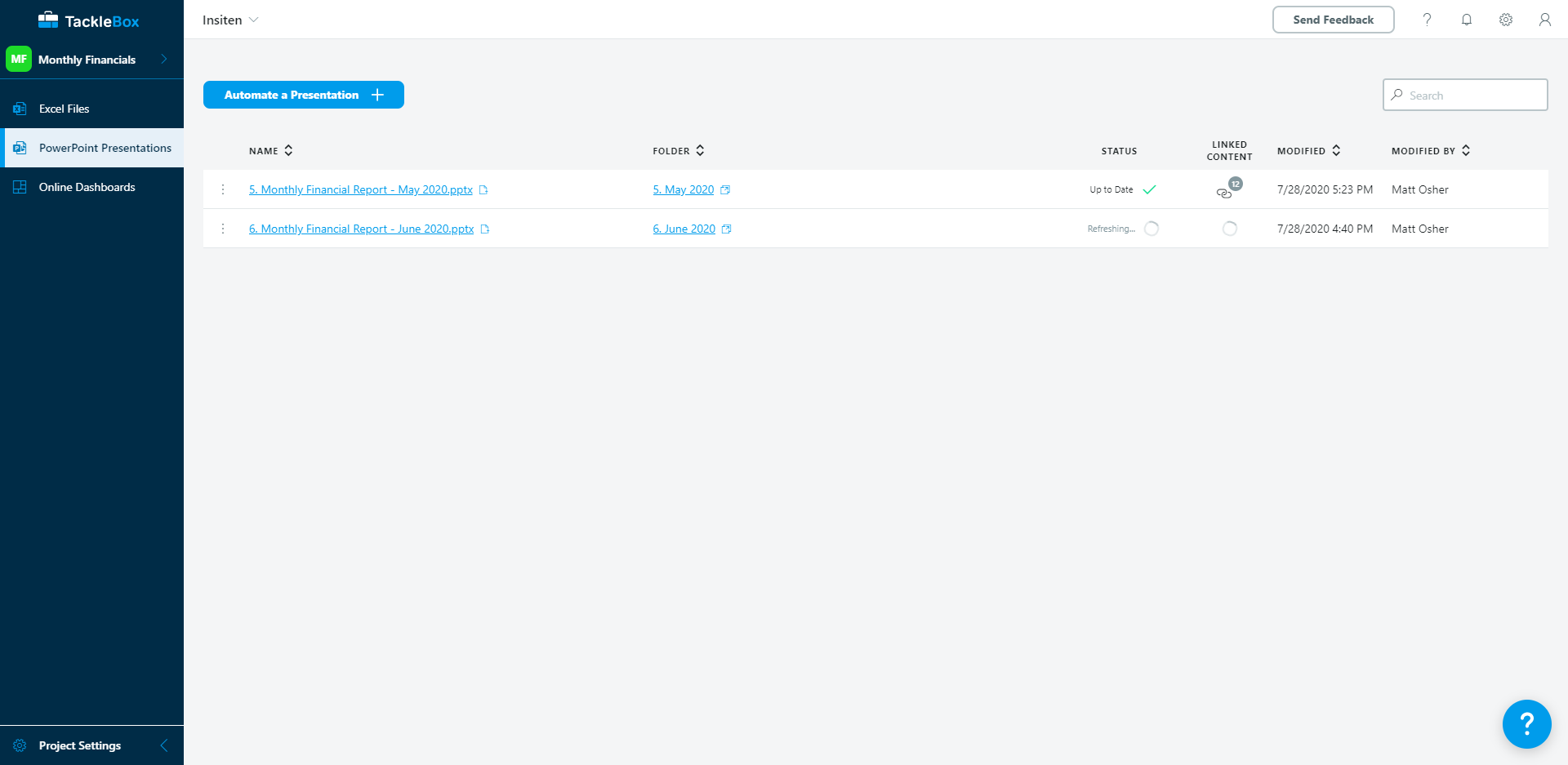This image depicts a digital interface titled "Tackle Box" in the upper left-hand corner. It features a sidebar with a section labeled "Monthly Financials." Within this section, there are categories for "Excel Files," "PowerPoint Presentations," and "Online Dashboards," with the "PowerPoint Presentations" category highlighted.

To the right, two PowerPoint presentations are listed—one dated May 5th, 2020, marked as "Up to Date," and another from June 6th, 2020. Each entry includes the date and time they were last modified, along with the name of the person who modified them. These presentations are monthly financial reports for May and June of 2020.

The Tackle Box appears to function as a repository for storing, accessing, and reviewing various digital files such as presentations and reports. 

At the bottom of the sidebar, there is an option labeled "Project Settings." In the upper right-hand corner of the interface, several icons are displayed: a feedback button, a question mark for help, a bell indicating notifications, a settings button, and a profile button for the logged-in user.